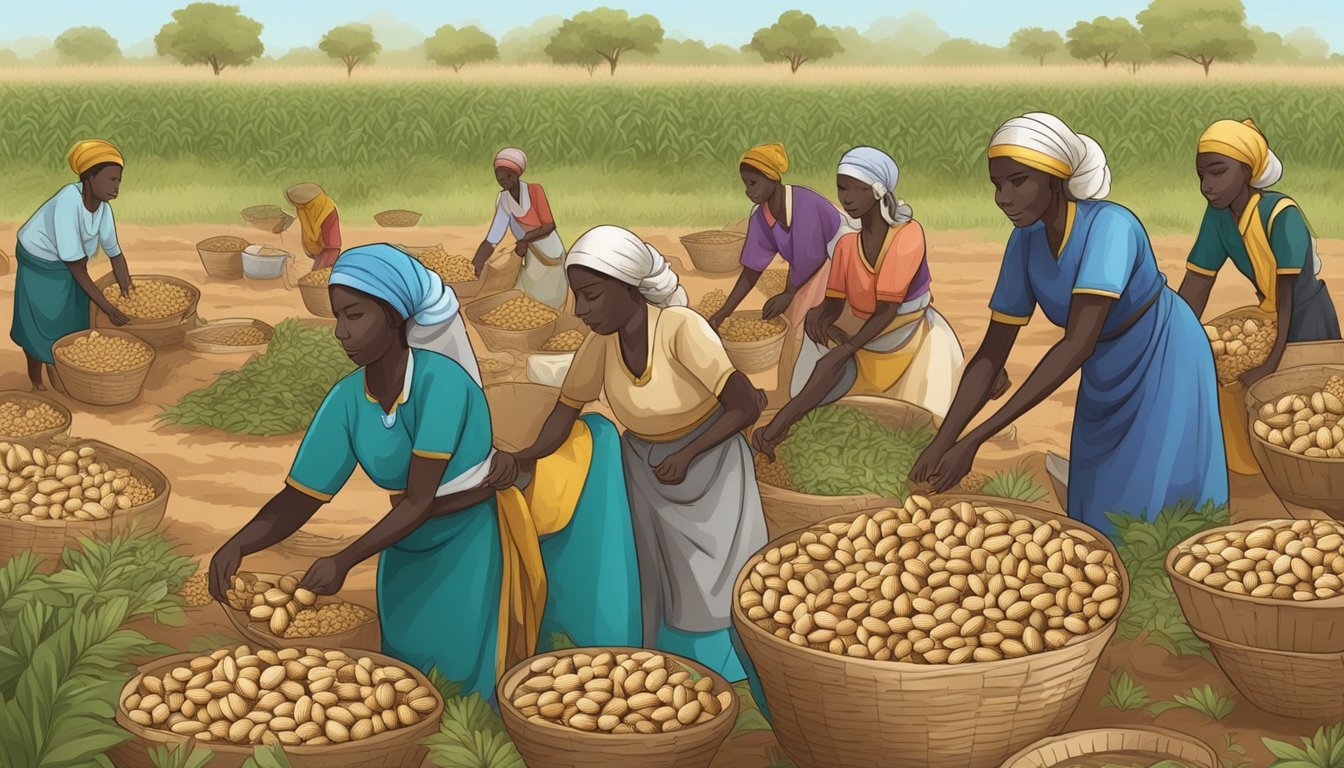This AI-generated illustration portrays eight black women diligently engaged in agricultural activities, seemingly harvesting and sorting potatoes or a similar brown, nut-like fruit. Each woman is dressed in brightly colored attire, ranging from dresses in hues of blue, purple, and mixed colors to brightly colored shirts and skirts, appropriate for hot weather. They also wear head coverings that hold their hair back as they work. The women are depicted with their heads down, fully focused on the task at hand, placing their hands into baskets filled with the produce, which varies in size and some appear to include leafy plants. The image, viewed from the front, has a sense of depth with a background showcasing a field that might resemble corn stalks, tall grass, and an array of trees under a blue sky. The illustration presents an uncanny, slightly malformed depiction of limbs and eyes, characteristic features of AI-generated art.